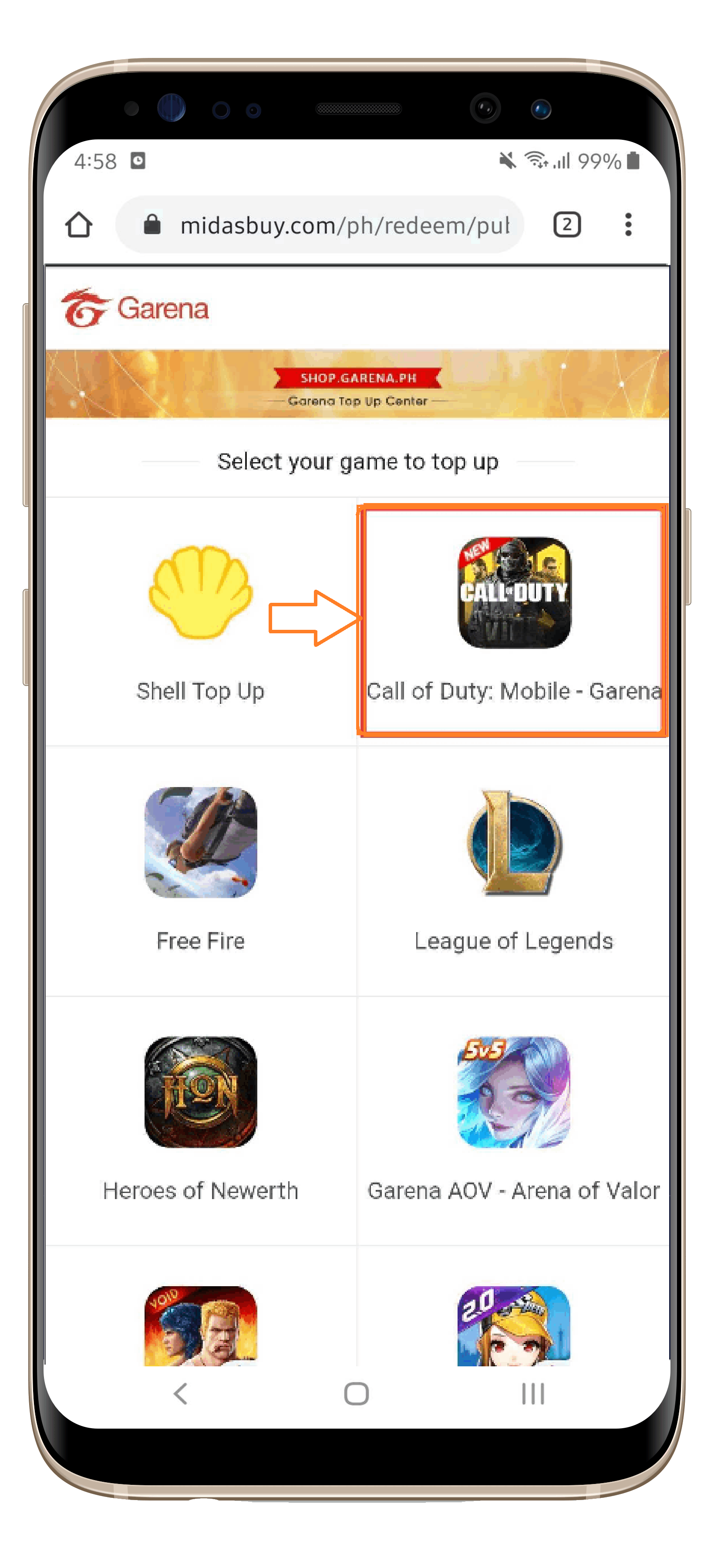The image depicts a screenshot of a mobile phone displaying a website. The mobile phone is black with a silver border, featuring two buttons on the left side and one on the right. The screen shows a website with a white background, captured at 4:58, with the battery at 99% charge. The URL bar indicates the website address as Midasbuy.com/ph/redeem/pul.

Beneath the URL, the website is branded as "Garena," with its name in red and an icon resembling a red eye. An orange banner spans across the page, possibly depicting a cityscape, with the text "shop Garena.ph" in a red section and "Garena Top Up Center" prominently displayed. Below this banner, in black text, is the instruction "Select your game to top up."

The website layout includes two columns, each showcasing four games, listed from top to bottom and left to right. The games are:

1. Shell Top Up, represented by a yellow shell icon.
2. Call of Duty Mobile.
3. Garena Free Fire.
4. League of Legends, symbolized by a large "L."
5. Heroes of Newerth.
6. Garena AOV (Arena of Valor).
7. An unidentified game with an image of a woman with blue hair alongside a muscular bald blonde man.
8. Another unidentified game featuring an anime character.